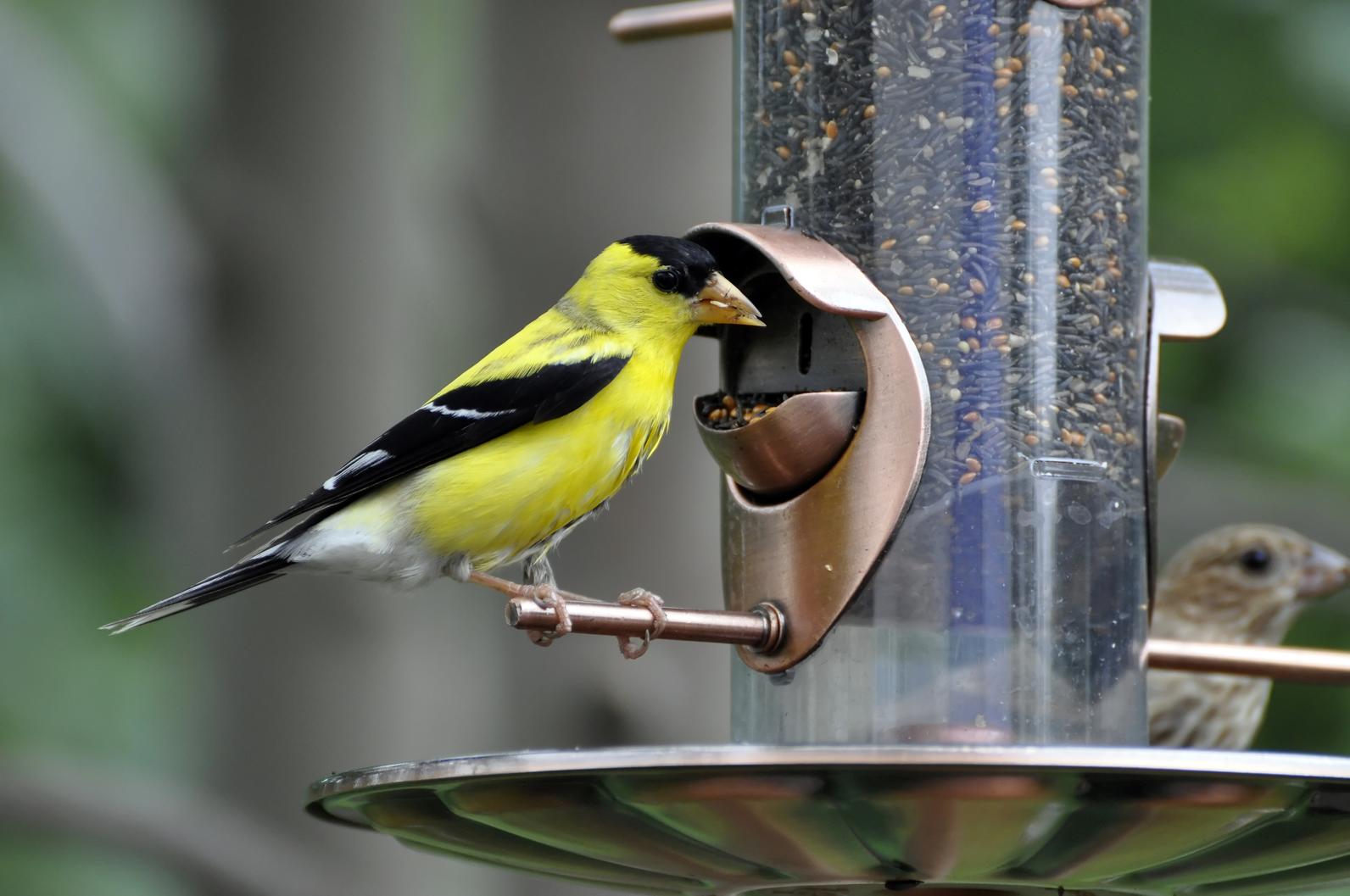The image showcases a vibrant bird feeder scene with two distinct birds. The central focus is a striking bird with a yellow underbelly and upper body, complemented by black wings adorned with a white streak, and a black head. The bird's beak is a neutral brownish-yellow color, and it stands on a perch with pink feet, feeding from a spout section of the feeder. The bird feeder itself has a clear glass exterior, showcasing a mix of mostly black seeds, interspersed with yellow kernels and gray seeds. The feeder appears to have a bronze or copper feeding section and an integrated birdbath underneath to catch excess seeds. On the opposite end of the feeder, a brown bird with a prominent black eye peers into the distance. The background features a blurred array of green leaves and trees, creating a natural outdoor setting. The photo captures a serene moment in nature with detailed observations of both birds and their shared feeding space.